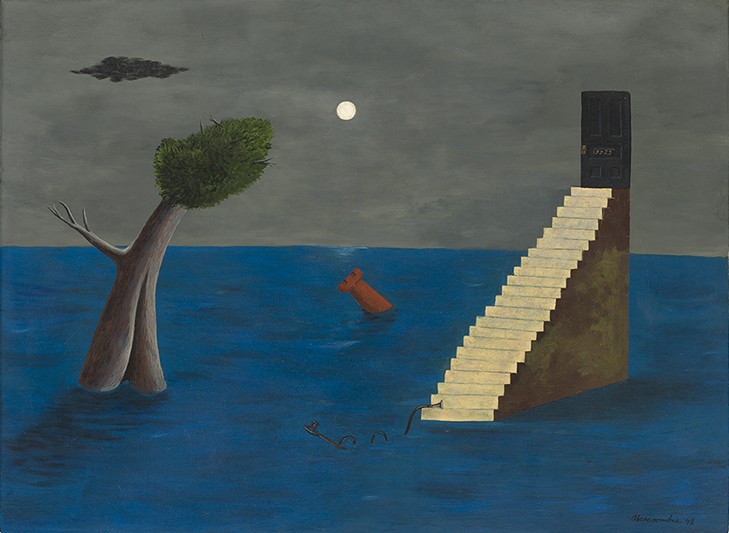This detailed and surrealistic painting by Gertrude Abercrombie features an abstract depiction combining various fantastical elements. Set during nighttime, the lower half of the image showcases dark blue water, giving a deep and immersive feel. A set of yellowish-brown stairs ascends from this ocean, prominently 3D in nature and steep, leading to a solitary brown door that stands against a backdrop of a hazy gray sky. The staircase seemingly leads nowhere, as water and sky extend unbounded behind it. 

To the left of the staircase, a tree that resembles a person's body stands with its branches extending left, the top curving toward the center, adorned with a circular bush-like foliage reminiscent of a person’s hair. Above this tree, a lone black cloud floats in the sky, enhancing the surreal atmosphere.

The centerpiece of the water holds a striking red rook chess piece, leaning diagonally and appearing to float. Dominating the sky is a small, glowing white moon placed centrally, providing a serene contrast to the abstract elements below. Lastly, at the base of the stairs, a black stick figure with an appendage over the bottom step adds an enigmatic touch to this modern abstract work.